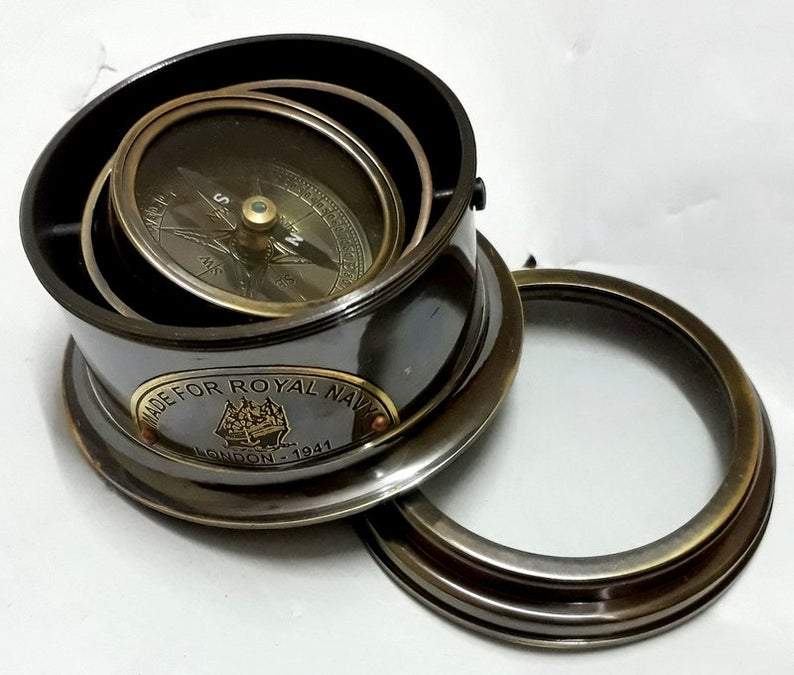The image captures a vivid, close-up color photograph of an antique compass, meticulously crafted in a distinctive conical shape and carefully opened to reveal its detailed components. The compass, which is primarily dark brown with a reflective metallic finish, rests at a slight angle atop its upside-down lid. Prominently stamped on the front in bold black and gold lettering is "Made for Royal Navy" in an arc, accompanied by an intricate emblem of a ship, and below it, the inscription "London-1941."

The compass itself is intriguingly designed with a hollowed-out structure, mounted on a horizontal bearing rod that is visibly riveted to the casing, allowing it to tilt slightly to the right. Its face showcases a bronze hue with elegant gold detailing, accentuated by a glossy surface. Though partly obscured, the inner workings reveal intricately positioned hands and notches. 

The entire setup, including the precision of the craftsmanship and historical inscriptions, suggests a vintage appeal, likely intended for product advertisement. Encasing the compass, the small circular box features a clasping ring at the bottom, designed to keep the pieces securely together when not displayed. This exquisite piece is set against a marble-like white surface with subtle grey striations, enhancing its antique allure.